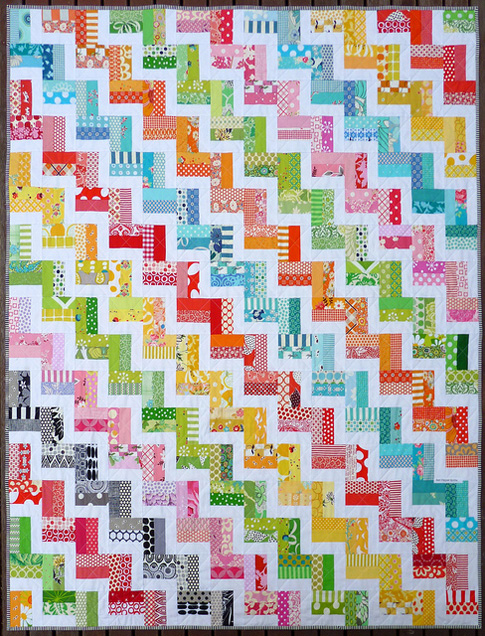The image features a colorful, intricate pattern reminiscent of a quilt or a painting, framed by a thin black border. Running diagonally from the top left to the bottom right corner are prominent white zigzag lines, sectioning off various rectangular color blocks. Each vibrant section is filled with detailed, smaller patterns in shades of blue, orange, green, pink, red, yellow, and black. The colors are repeated in descending order from the top left: green, red, yellow, blue, pink, green, orange, blue, red, yellow, green, pink, black, red, and orange, with each block neatly separated by the thick white zigzag lines.